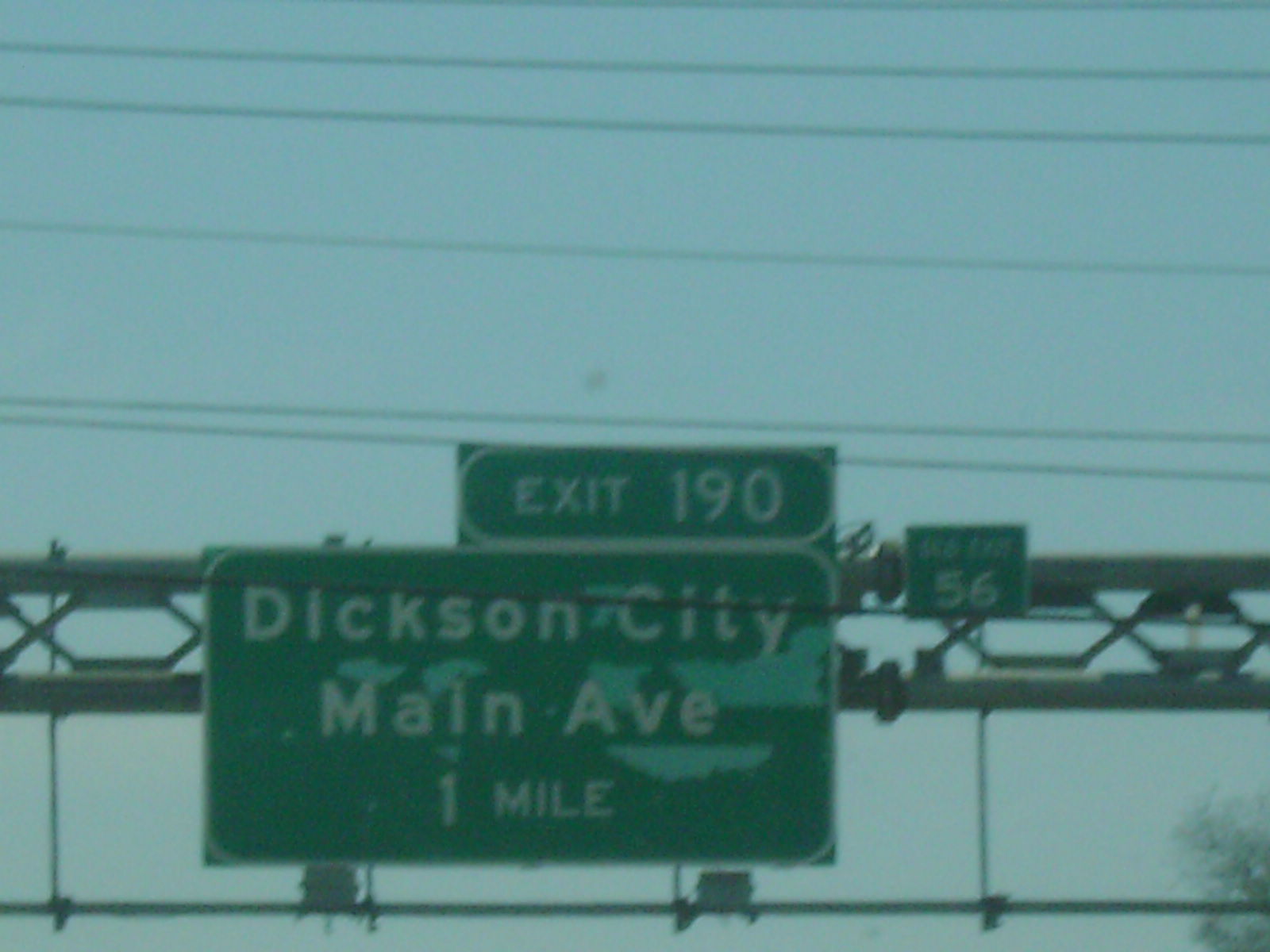This photograph captures an overhead highway sign supported by a sturdy steel frame. The sign is primarily green with crisp white text for optimal visibility. The upper right section of the sign features a smaller, rectangular plaque that indicates "Exit 190" in bold lettering. Below this, the larger green sign provides navigational information, reading "Dixon City Main Avenue 1 mile." The entire structure is accentuated by the presence of power lines running above it, adding to the urban roadside atmosphere.